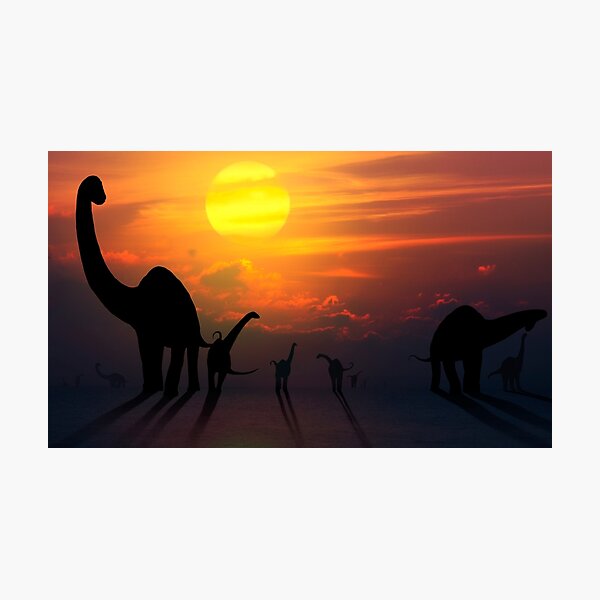A vivid and artistic print titled "Sauropod Sunset" depicts a prehistoric scene at dusk. The composition features a gradient sky transitioning from a brilliant orange near the horizon to hues of yellow, pink, and bright purple higher up. The sun, a fully visible yellow orb, sits slightly left of center above a layer of clouds that darken to black at the horizon and become puffier and streaked as they ascend. Silhouetted against this colorful backdrop, a group of sauropod dinosaurs with long necks and small heads are arranged in a line across the bottom of the image. The largest dinosaur is located in the bottom left corner, with progressively smaller ones trailing to the right. More dinosaurs, shrouded in a hazy fog, can be seen in the distance, contributing to the layered depth of the scene. Their black shadows stretch forward, grounding the ethereal quality of the vibrant sky above. The overall effect captures the majestic peacefulness of these ancient giants roaming beneath a glorious setting sun.